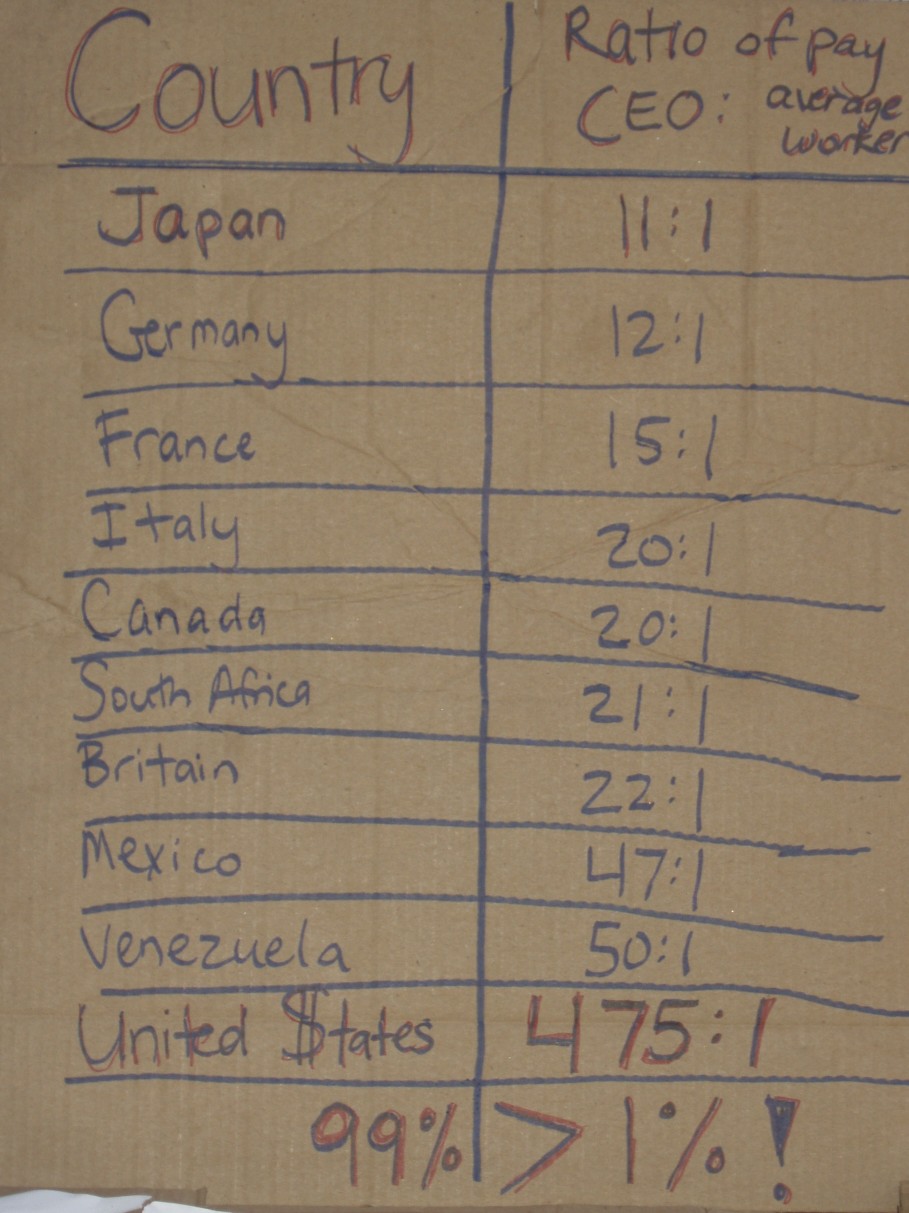The image depicts a scanned, handwritten chart on construction paper with a grid-like layout. It organizes information with two columns: the left column titled "Country," written in red and blue marker, and the right column labeled "Ratio of Pay (CEO : Average Worker)," also in red and blue marker. 

The chart lists the following countries and their respective CEO-to-average-worker pay ratios:

- Japan: 11:1
- Germany: 12:1
- France: 15:1
- Italy: 20:1
- Canada: 20:1
- South Africa: 21:1
- Britain: 22:1
- Mexico: 47:1
- Venezuela: 50:1
- United States: 475:1

The handwritten lines are slightly curved and jagged, suggesting the document was created manually. At the bottom of the chart, there is a notable text: "99% > 1%" accompanied by an exclamation mark, possibly indicating a protest message.